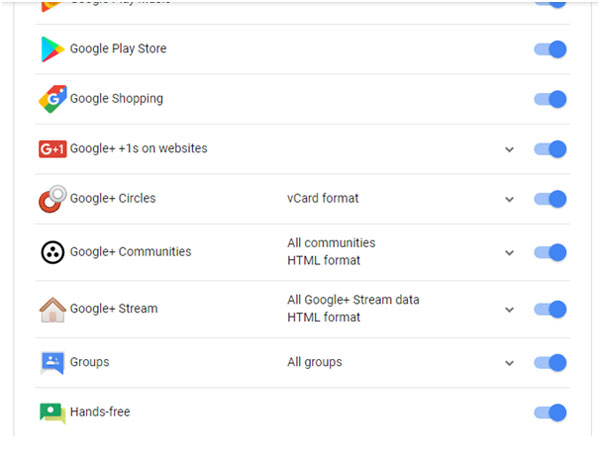The image depicts a settings page on a desktop computer, specifically for a Google-related service. The interface includes multiple toggle switches that allow the user to enable or disable various features for display on a website. Here's a detailed breakdown of the elements depicted:

- A section titled "Streaming Service of Google Play TV" allows toggling on or off all Google Play Store features.
- Another toggle switch controls whether all Google Shopping features are enabled or disabled.
- There is a feature labeled "Google+1s on Websites" with a drop-down menu and a toggle switch to turn it on or off.
- The "Google+ Circles" feature is presented in a card format with an additional drop-down menu and a toggle switch.
- "Google+ Communities" are listed with an HTML format option, accompanied by a drop-down menu and a toggle switch.
- The "Google+ Stream" data is also available in HTML format, featuring a drop-down menu and a toggle switch.
- The section titled "All Groups" includes a toggle switch for enabling or disabling all groups, along with a drop-down menu.
- Finally, there is an option labeled "Hands-Free" without a drop-down menu but with a toggle switch to enable or disable the feature.

The layout appears extensive and detailed, suggesting it is designed for a desktop computer rather than a phone screen.